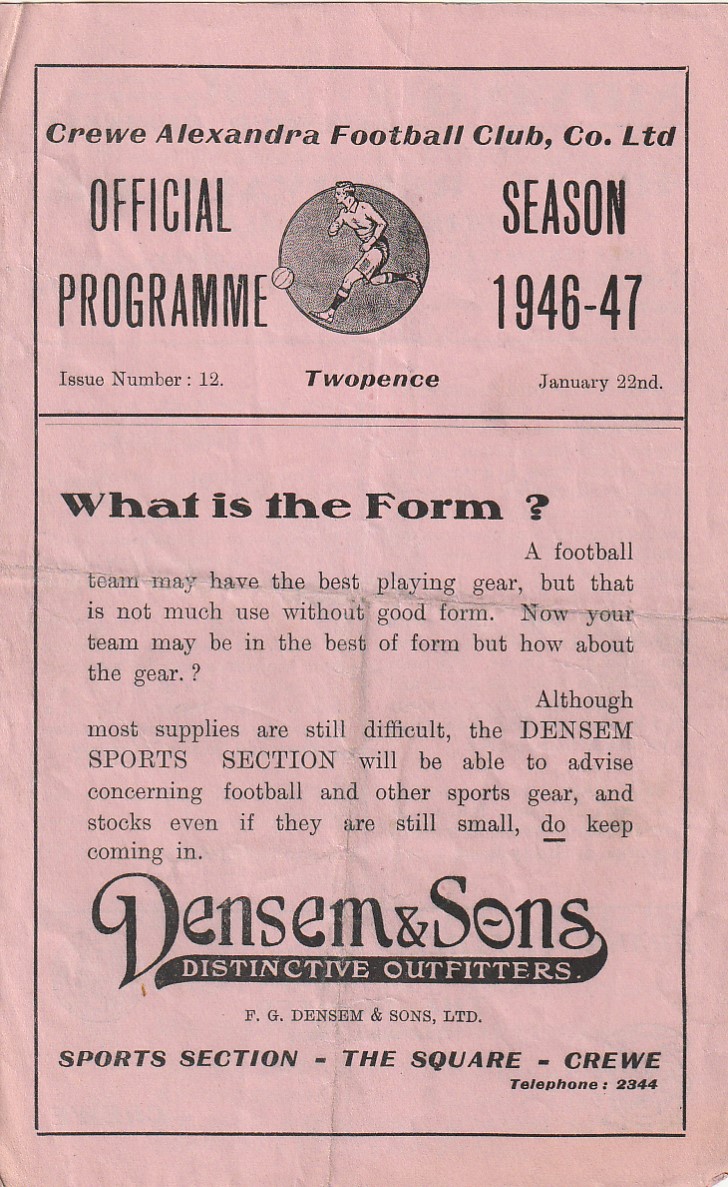This image depicts a vertical, rectangular, and crinkled, dusty-pink newspaper clipping or booklet page, featuring a pinstripe border. The top section is labeled "Crew Alexandra Football Club CO.LTD" in black print. Below it, the text reads "Official Program, Season 1946-47," flanked on the left by "Issue Number 12" and on the right by "January 22nd." A central black circle contains an illustration of a man in a uniform about to kick a ball. The program is priced at "2 pence." 

The bottom section poses the question: "What is the form?" followed by, "A football team may have the best playing gear, but that is not much use without good form. Now your team may be in the best of form, but how about the gear? Although most supplies are still difficult, the Dentson Sports Section will be able to advise concerning football and other sports gear and stocks, even if they are still small, do keep coming in." 

The final lines provide business information: "Dentson & Sons, Distinctive Outfitters, FG Dentson & Sons LTD, Sports Section-Square-Crew, Telephone 2344."